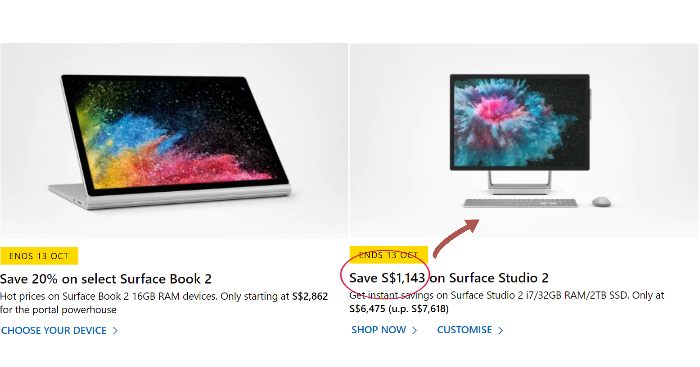The image presents a promotional side-by-side comparison of two Microsoft devices: a laptop on the left and a desktop monitor on the right.

On the left, the laptop is identified as the Surface Book 2 and is highlighted with a yellow box indicating the promotion ends on October 13th. Below this box, it features a sale offering a 20% discount on select Surface Book 2 models. Specifically, the Surface Book 2 with 16GB of RAM is promoted, starting at a price of $2,862, marketed as the "Portal Powerhouse."

On the right, the desktop monitor is the Surface Studio 2, also with a promotional notice ending on October 13th. This device is advertised with a significant discount of $1,143. It highlights the Surface Studio 2 with an i7 processor, 32GB of RAM, and a 2TB SSD, available at a price of $6,475, marked down from $7,618. 

The image includes two call-to-action buttons: "Shop Now" on the left under the Surface Book 2, and "Customize" on the right under the Surface Studio 2.